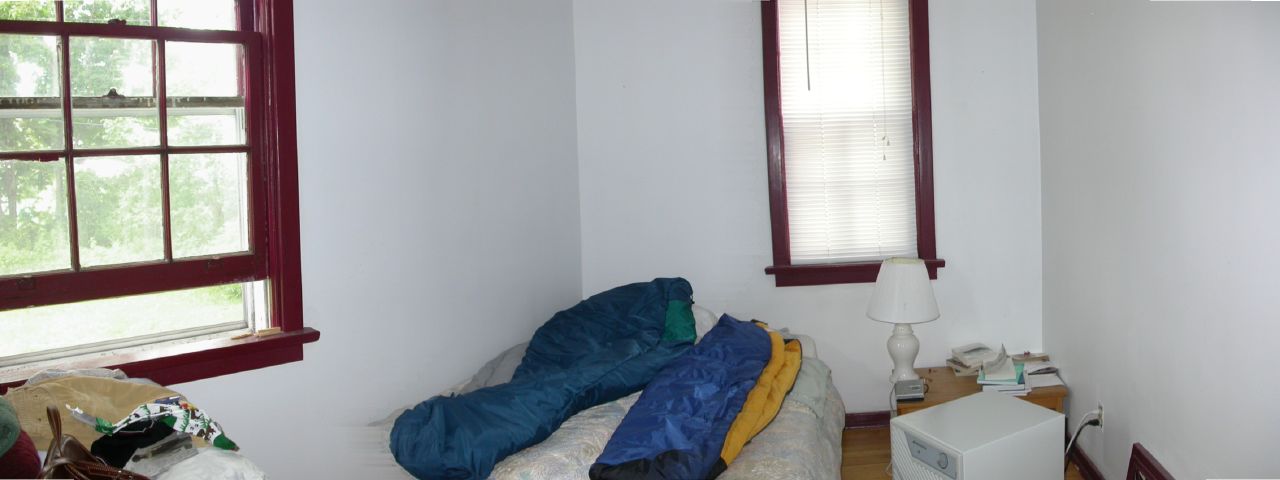This image depicts a small and narrow bedroom with white walls and two windows framed in dark brown wood. The bed, which lacks a frame, is positioned against the back and left walls, covered with two blue sleeping bags—one revealing a yellow interior. To the right of the bed, there is a modest brown end table cluttered with paperwork and topped with a white lamp. Nearby, a computer base and a white box are visible. The back wall features a skinny window with its shades down, while the larger window on the left wall, partially hidden and partially open, exposes a view of tree leaves. A pile of clothes rests on the floor at the bottom left of the image.